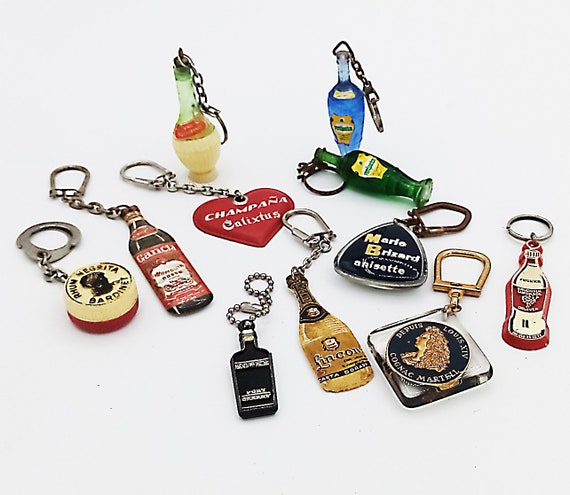A diverse collection of keychains, predominantly shaped like bottles, is organized in the image. At the top, two bottles stand upright with keychains attached to their lids; one is blue while the other is green with a yellow base. Below these, in the middle, a silver chain hangs from a red heart-shaped keychain that reads "Capana Calictus" in white letters.

To the left of the heart keychain, a flat bottle with a red label rests on the ground. Adjacent to it lies another bottle with a circular label resembling a handcuff, white on top and red on the bottom. At the very bottom, a dark black bottle and a light gold bottle are positioned next to each other. Nearby, a square silver keychain encloses a black coin featuring a woman’s face.

On the far right side, there is a keychain resembling a ketchup bottle, red with a white label in the center. Centrally located is a guitar pick-shaped keychain, silver with a black interior, that reads "Mario, record, and see it in the middle" accompanied by a rusted chain.